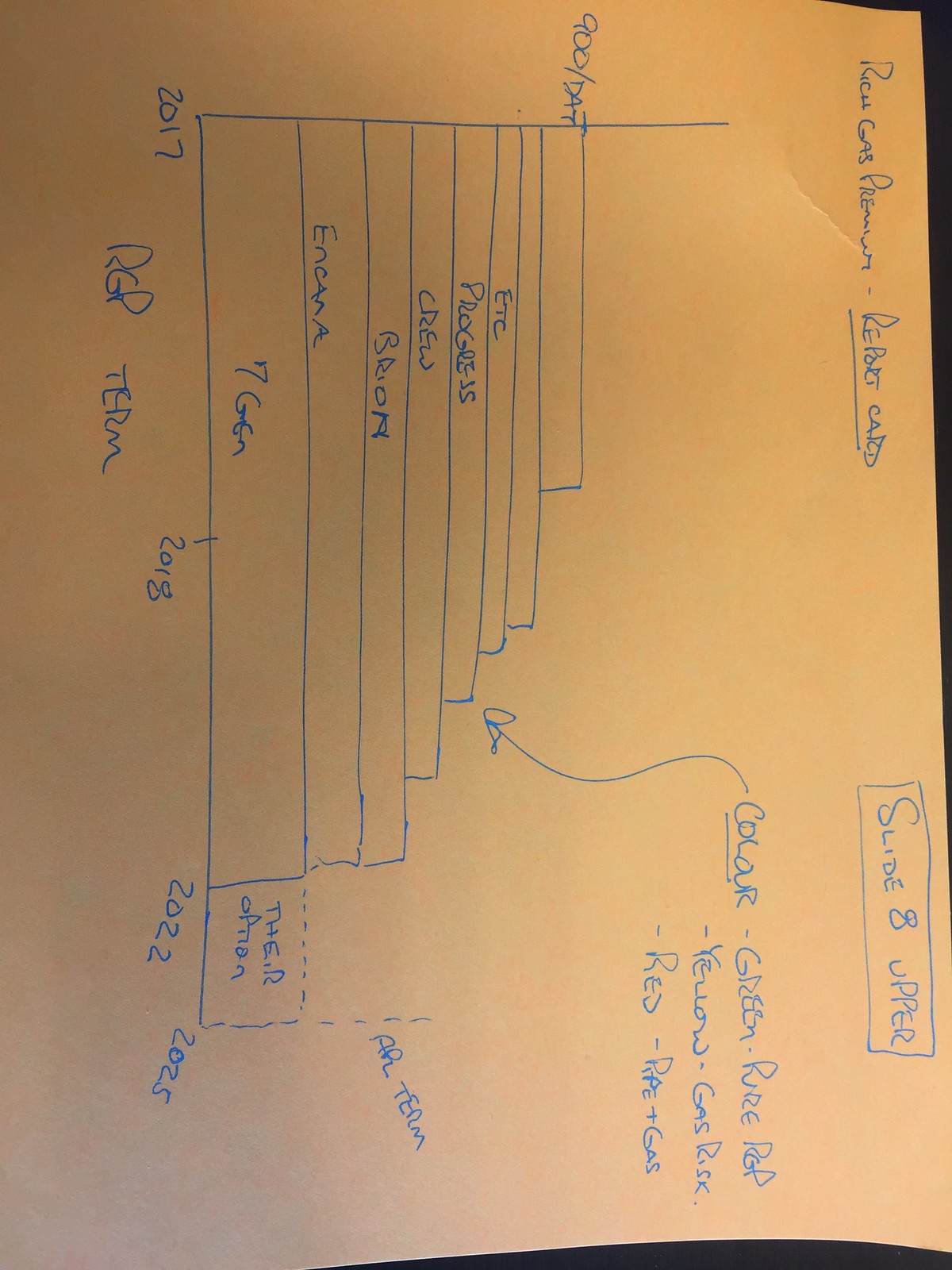This image is a photograph of a detailed, hand-drawn chart on gold-colored paper, oriented on its side, making the text difficult to read. The chart, created with blue ink, is rich with information despite the challenging legibility. In the upper left corner, the title "Rich Gas Premium Dash Report Card" is prominently displayed and underlined. To the top right, encased in a box, is the label "Slide 8 Upper." Below this, there's the word "Color" underlined, with an arrow pointing downward towards a graph. This graph, central to the chart, uses the colors green, purple, red, and yellow to denote different categories or levels. Labels include terms such as "Gas Risk" and "Red RPE Plus Gas."

The graph itself appears to be a progression chart, resembling a stairway, with categories like "Progress," "Crew," "7 Gen," "ENCAA," and "BRON" arranged in ascending order. Key time points noted on the chart are 2017, 2018, 2022, and 2025. This chart captures a sequence of events or metrics, documenting changes or development phases over time, making it a comprehensive yet intricate depiction of data related to gas and associated risks.